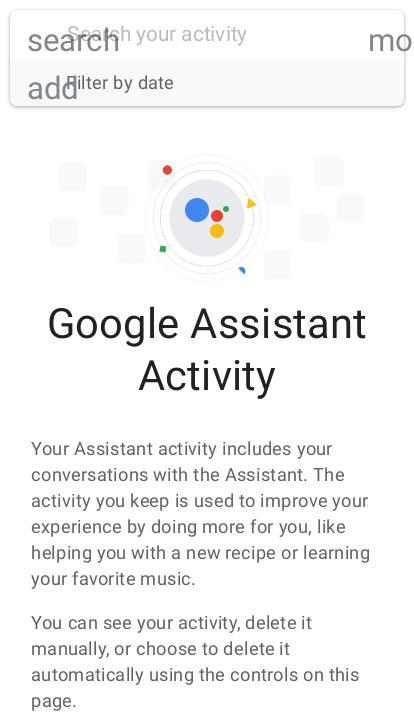In this image, the top section features text options including "Search your activity," "Search," "Add," and "Filter by dates" against a white background. The middle portion is dedicated to "Google Assistant Activity," explaining that your Assistant activity includes conversations with the Assistant. This activity enhances the user experience by providing personalized assistance, such as finding new recipes or learning your favorite music. Users can view their activity, manually delete it, or set it to auto-delete using the controls provided on the page. The text is displayed in black, and the overall design incorporates Google’s signature colors of red, blue, green, and yellow. The image also includes various shapes like circles, squares, triangles, and semicircles, adding to the visual appeal.